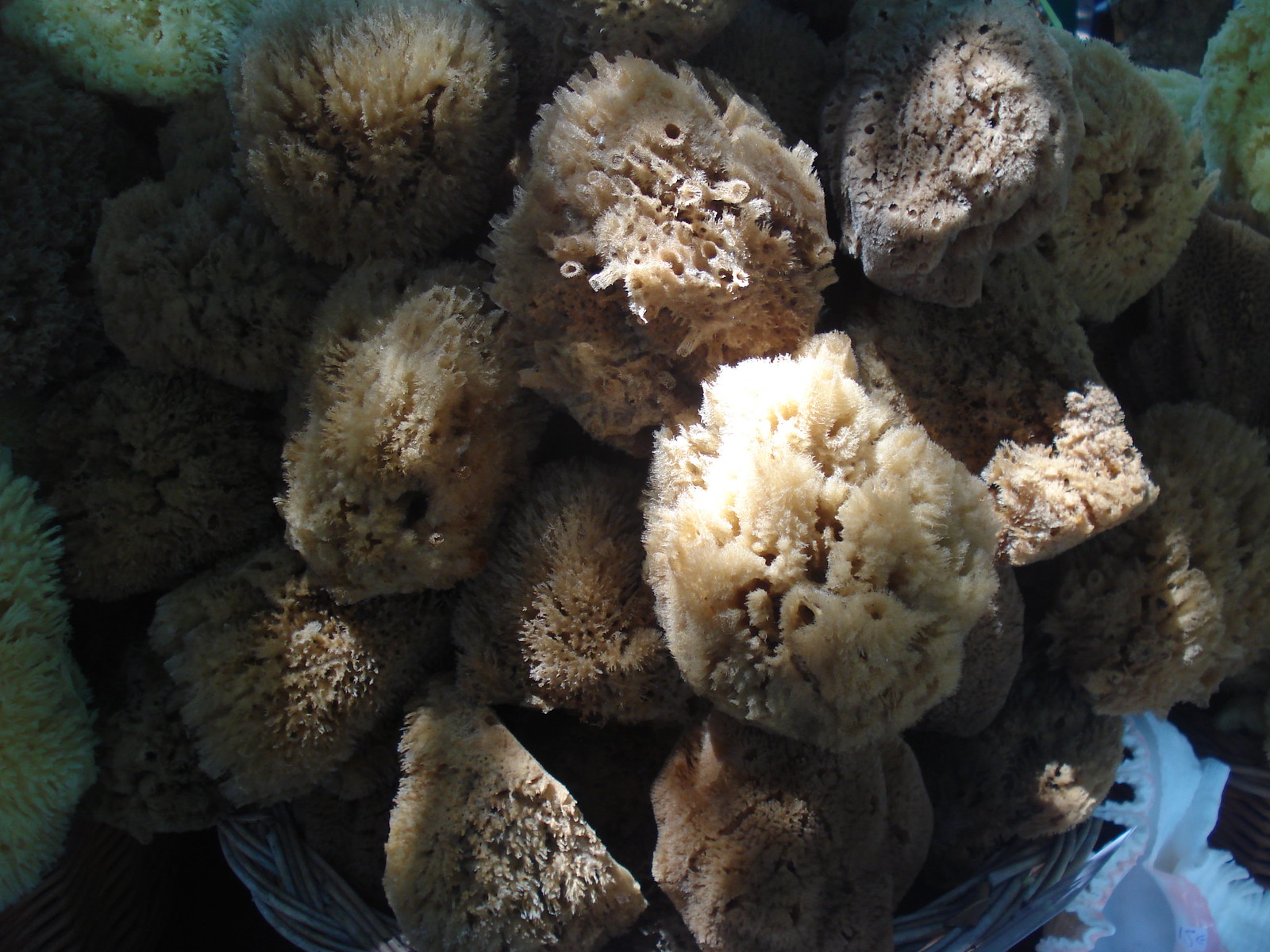This is an underwater color photograph focusing on a dense aggregation of coral, capturing the spectacular diversity of a coral reef. The main subject is a cluster of approximately 15 to 20 coral pieces tightly packed together, forming a visually striking mass. Each coral piece is roughly the size and shape of a basketball, sporting a range of brown tones from tan to yellowish to cocoa, and they all possess a distinct fuzzy texture. The sunlit water is clear, revealing vibrant, illuminated colors. Notably, there are pockets of other corals on the periphery: green and yellow-hued corals inhabit the top left and top right corners, while similar shades are visible on the bottom left. In contrast, the bottom right corner features a distinct bluish illumination, potentially indicating a different organism or coral type, such as a jellyfish. The scene is likely set on or near a reef, with hints of yellowish or off-white structures providing a backdrop to the stunning, diverse coral display.